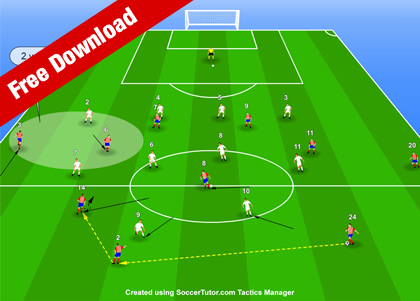This image is a digital rendering from a computer program, most likely an advertisement for a football tactics application called SoccerTutor.com Tactics Manager. It shows an overhead view of a bright green soccer field with alternating dark green stripes, suspended in a light blue background. On this field, players are depicted in red jerseys with blue shorts and white jerseys. Numbers are displayed above them, and they are connected by various lines—black directional lines and dotted yellow lines—illustrating complex football strategies. In the middle of the field, a white circle and another filled circle off to the left indicate tactical points of interest, where players are actively converging around the ball. In the top left corner, a red rectangle banner states "free download" in white letters. At the bottom of the image, it reads "created using SoccerTutor.com Tactics Manager," identifying the source of this tactical diagram. Additionally, a white soccer goal outline is visible at the top of the image.